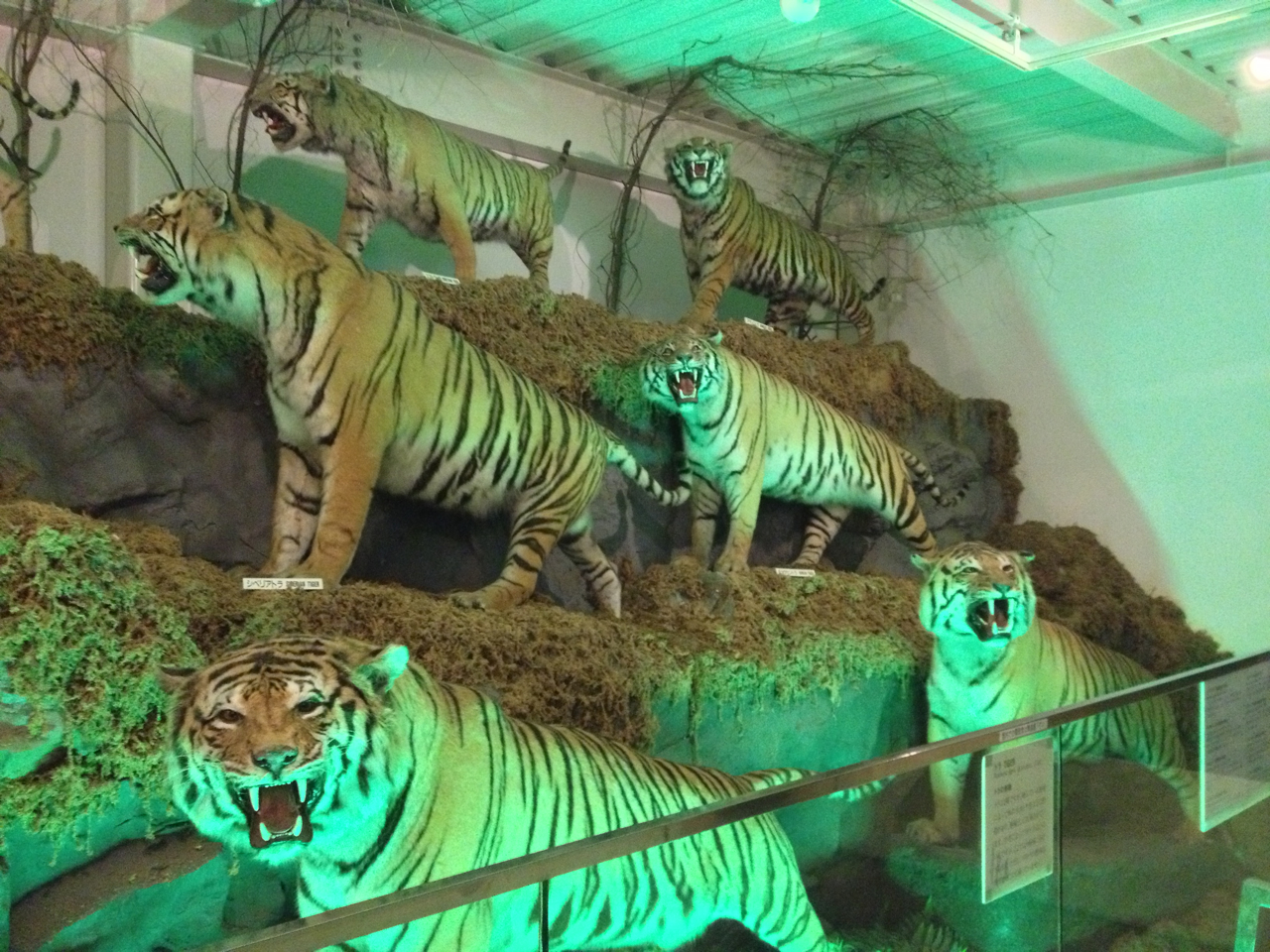The image shows a strikingly realistic exhibit in a museum or similar indoor space, featuring six meticulously arranged taxidermy tigers. The tigers, appearing almost lifelike, are displayed in three stepped levels on an artificial rocky landscape dotted with moss and scrubs. Each tier has two tigers that are posed with their mouths open in a menacing snarl, exposing their sharp canines. The exhibit is illuminated with a greenish light, enhancing its eerie atmosphere, and is housed within a room supported by steel beams and a corrugated ceiling, which also contributes to the green hue. The display is protected by a glass and steel barrier, topped with metal edging, ensuring visitors remain on one side. Each tiger is accompanied by a small white sign with labeling, possibly in an Asian language, providing additional information. The overall scene is both captivating and unsettling, creating a vivid and intense viewing experience.